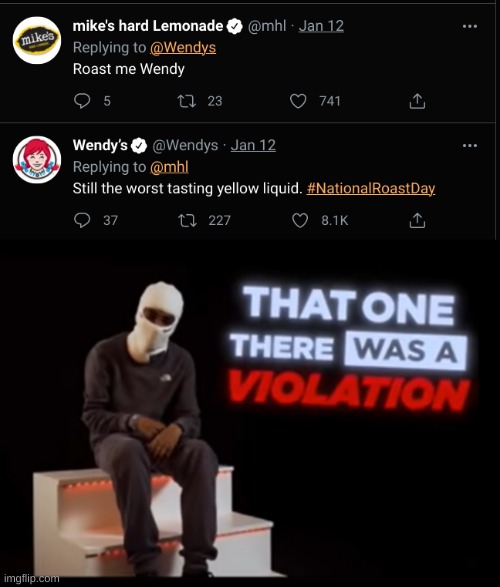**Caption for Social Media Post on X:**

In honor of #NationalRoastDay, a witty exchange between **@MikesHardLemonade** and **@Wendys** lights up our feeds. The verified account for Mike's Hard Lemonade cheekily challenges Wendy's with a tweet: "Roast me, Wendy." Wendy's, never one to shy away, delivers a scorching reply: "Still the worst tasting yellow liquid." 

Below the sharp-witted banter, an image commands attention. A Black man sits on two white, track-lit steps glowing with red illumination beneath each step. He's in a contemplative pose with his arms resting limply on his lap, gazing out from behind a full-face mask that reveals only his eyes. Dressed in a dark gray sweatshirt, matching sweatpants, and brown shoes, he epitomizes a cool, unbothered vibe.

Emphasizing the comical punch of Wendy's roast, bold text to his right declares: "That one there was a violation." The phrase is artistically presented with "That one there" in white, "violation" in red, and "was a" in gray set against a white background. 

This dynamic post captures the essence of digital humor and the unfiltered spirit of social media interactions.